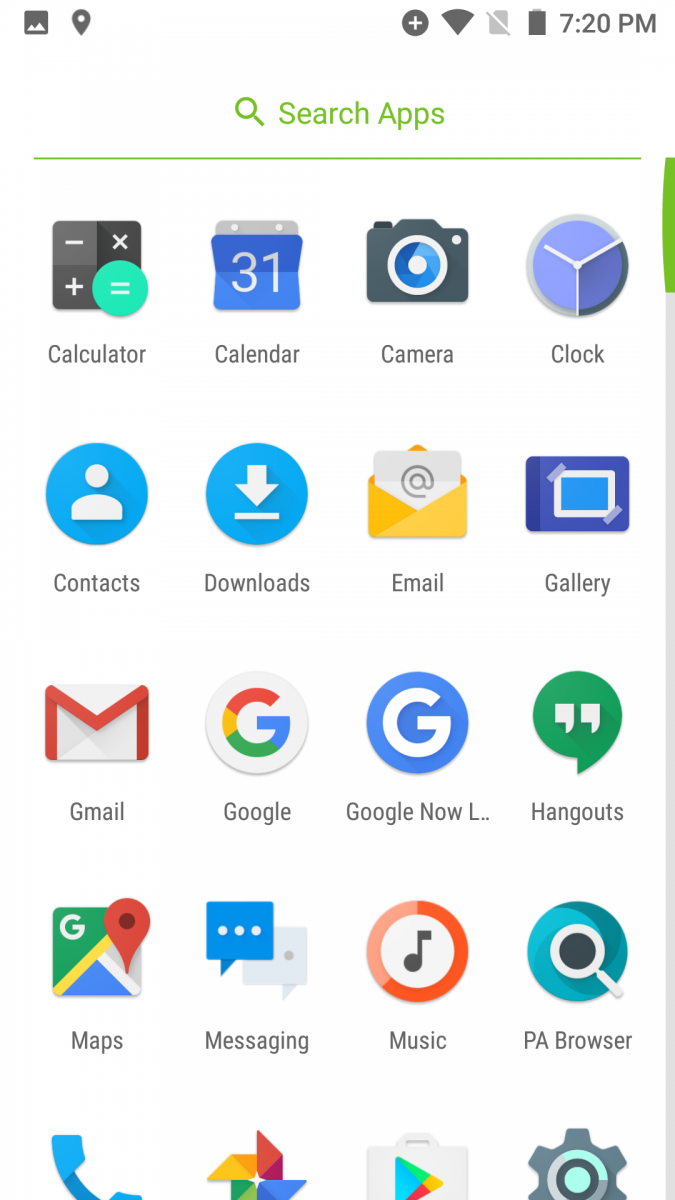Screenshot of an Android Phone's Extended App Screen

The image features a white background displaying the extended app screen of an Android phone. At the very top, a status bar shows several small icons from left to right: a location icon, a screenshot icon, a Wi-Fi icon, a mobile signal icon, a battery icon, and the time displayed as 7:20 PM. Beneath the status bar, the text "Search apps" is shown in green, accompanied by a magnifying glass icon to its right. A horizontal green line separates this section from the app icons below.

The screen showcases a grid of app icons, each consisting of an image and the corresponding app name underneath. The first row of apps includes Calculator, Calendar, Camera, and Clock. The second row features Contacts, Downloads, Email, and Gallery. The third row lists Gmail, Google, Google Now, and Hangouts. The fourth row displays Maps, Messaging, Music, and PA Browser. The fifth row is partially cut off but visible icons indicate Phone, Google Photos, Play Store, and Settings.

This descriptive caption captures the essential details and layout of the screenshot, providing a comprehensive view of the Android phone's app screen.